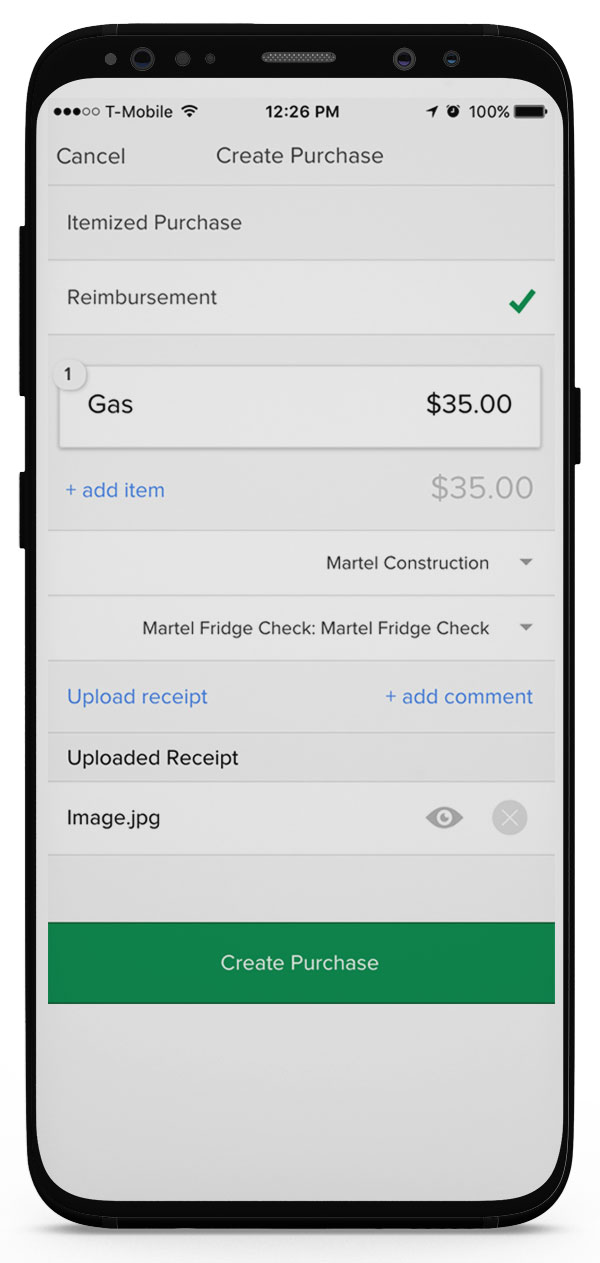The image depicts a smartphone screen showcasing an accounting app interface. In the top left corner, the carrier "T-Mobile" is displayed, followed by the Wi-Fi strength indicator showing three out of five circles. At the center of the upper bar, the time reads "12:26 p.m.", and the battery level is fully charged at 100%.

The screen is focused on a section of the app titled "Create a Purchase". Positioned in the top left corner of the application is the word "Cancel". Below, continuing to the right side, there is a green check mark next to the label "Reimbursement". Below this, an entry lists "Gas for $35" attributed to "Martell Construction", specifically noting "Martell Fridge Check".

At the very bottom of the screen, a prominent green button with white lettering reads "Create Purchase". Additional interactive sections feature blue text: "Add a Comment" with a plus sign, "Add an Item" with a plus sign, and "Upload Receipt". These elements suggest options to further detail or document the purchase entry.